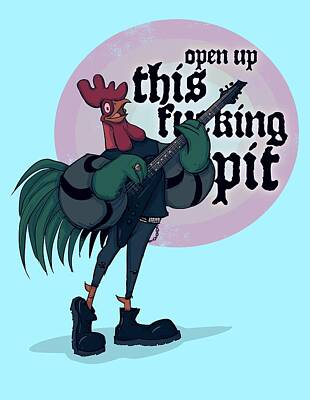The image is a detailed cartoon drawing featuring a humanoid rooster playing a guitar. The background is a light greenish-blue, with a large lavender circle in the center. Inside the circle, in black font, it says "Open up this fucking pit," though the rooster's guitar obscures the letter 'C' in "fucking," making it read as "flucking." 

The rooster stands on two legs, wearing an outfit consisting of a puffy gray jacket with mixed gray and black sleeves, blue skinny jeans, and black boots. It has green gloves on its hands, and its eye is bright white, while the beak is orange. The rooster's red comb and happy expression are prominent features, with its green tail feathers visible on the left side. 

The guitar has a V-shaped body, colored dark blue or black, and the rooster is actively strumming it, covering part of the text behind. Additionally, a black and silver belt with a chain is visible around the rooster's waist.